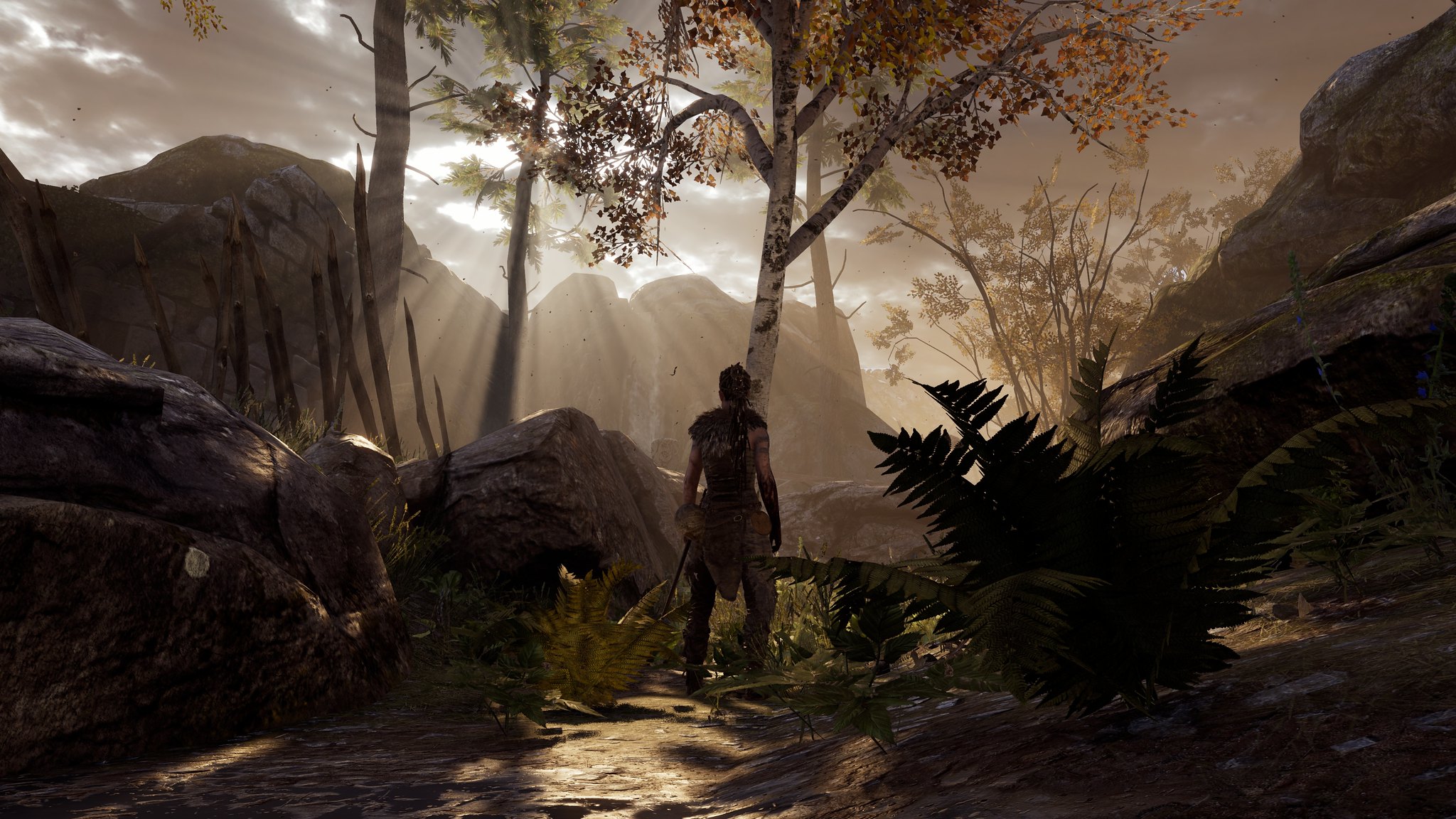In what appears to be a scene from a movie or video game, the central focus is a man viewed from behind, dressed in antiquated wilderness apparel reminiscent of traditional Indigenous garments. Feathers adorn his hair, and his bare arms are visible as he stands with one foot pointed forward, gazing intently towards the horizon. The foreground reveals a breathtaking natural landscape, featuring majestic mountains and clouds illuminated by piercing rays of sunlight. Surrounding the man is a lush wilderness teeming with trees, shrubbery, and rocky outcrops, adding to the scene's immersive, old-world ambiance.